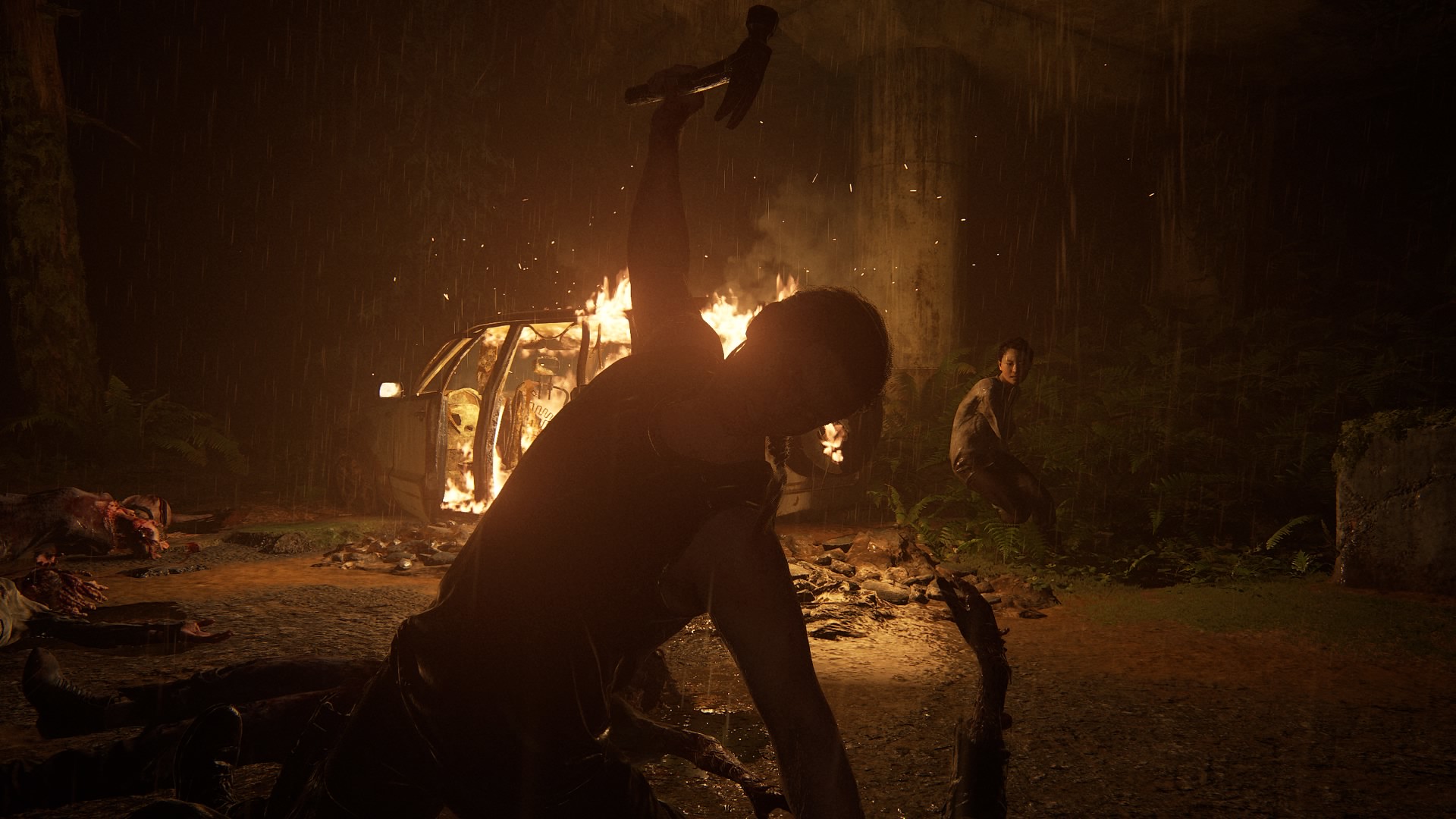In this highly realistic 3D-rendered scene, the focal point is a person poised in mid-action, about to swing a hammer down with immense force. The individual’s raised arm, clutching the hammer, suggests a moment of intense concentration, their gaze directed downward towards the viewer. Their other arm is extended out of the frame, gripping an unseen object.

The backdrop of this dark scene is a rugged, outdoor setting reminiscent of a makeshift campsite. The ground is a mix of dirt and scattered green foliage or rocks. Behind the central figure, another person is visible, observing the dramatic action. This onlooker stands near the charred, burning remains of a vehicle, now reduced to its fiery frame.

Further in the background, streaks resembling either a waterfall or vines cascading down from trees add to the eerie atmosphere. The predominantly dark environment is punctuated by the fire's harsh glow, casting striking silhouettes and sporadic spark effects that illuminate portions of the scene.

On the left side of the image, various indistinct objects are scattered on the ground, with faint details of surrounding plant life. This intricate composition combines elements of tension, destruction, and nature, captured through the dramatic contrasts lit by the fire.